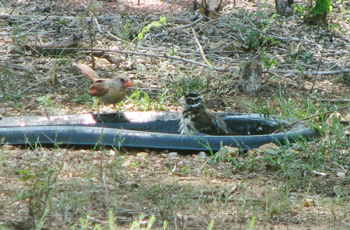The photograph presents an intriguing, somewhat blurry scene set outdoors in what appears to be a sparse, grassy field interspersed with sticks and smaller plants. At the center of the image is a black or gray plastic object—possibly a small boat, raft, or makeshift bird bath—that contains a small puddle of water. Perched on this object are two birds. One bird, which is brown and red with a long tail, stands along the edge, while the other, which has black, white, and tan feathers, and is possibly a baby cardinal with an orange beak, is situated in the center. The lighting in the photograph reveals patches of sunshine that cast shadows across the grassy field. The overall composition suggests a quiet moment in nature, despite the unclear, blurry quality of the photo.